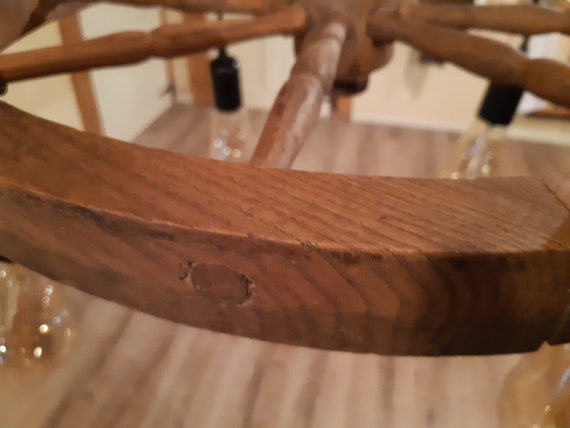In the image, we see a close-up view of what appears to be a circular chandelier made of dark brown wood. The chandelier features five evenly spaced wooden rods or spokes extending from the center to the edge, reminiscent of a wheel's structure. In the middle of the chandelier is a prominent circular mark. Hanging from these beams are several light bulbs set in black holders, with two clearly visible on both the lower right and lower left corners, and additional bulbs on the left and right sides. The background shows a light brown wooden floor, creating a warm, cohesive backdrop that complements the chandelier’s design. The clarity and magnification of the shot emphasize the intricate details of the chandelier’s wooden construction and the arrangement of its light bulbs. Some viewers also note what appear to be floating bubble-like objects near the bulbs, adding an extra layer of curiosity to the image.